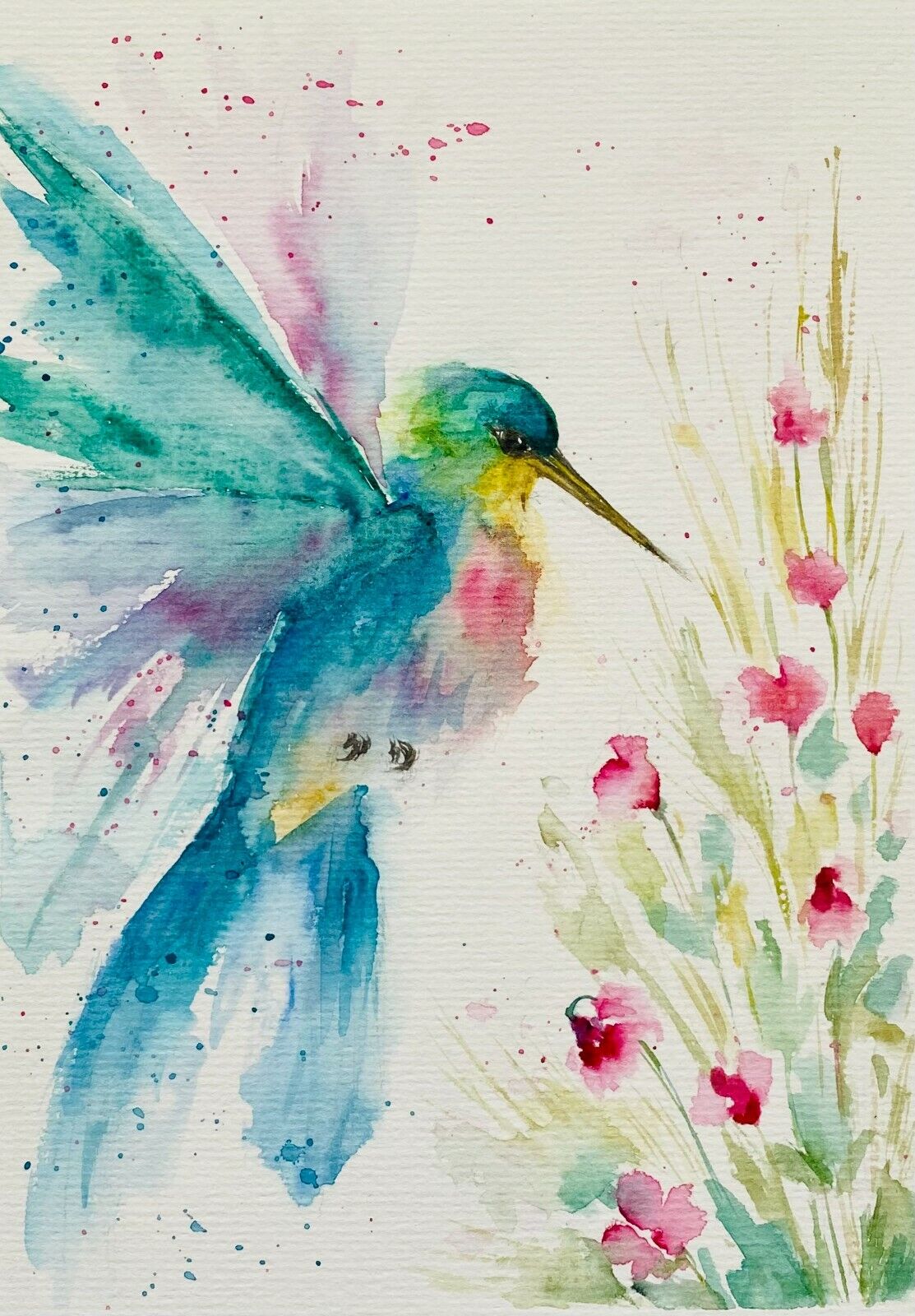This watercolor painting, possibly on cardstock, features a vibrant scene with a large, colorful hummingbird in mid-flight. The hummingbird, depicted with a blend of turquoise, aquamarine, teal, cyan, and pink hues, boasts a striking golden-yellow beak, dark black eyes, and bright yellow feathers on its chest. The bird's wings show dynamic brushstrokes that transition from strong and opaque by the body to more transparent at the edges, enhancing the sense of movement. 

To the right of the hummingbird is a sprig of flowers with an array of yellowish-green leaves and bright pinkish-red flower bulbs. The flowers are amidst grass stems, adding to the natural setting. The painting's background is subtly textured, typical of high-quality watercolor paper. Throughout the piece, there are artistic spatters of watercolor paint, with blue spatters near the bird and red and yellow across the flowers, adding a lively, painterly effect to the whole composition.